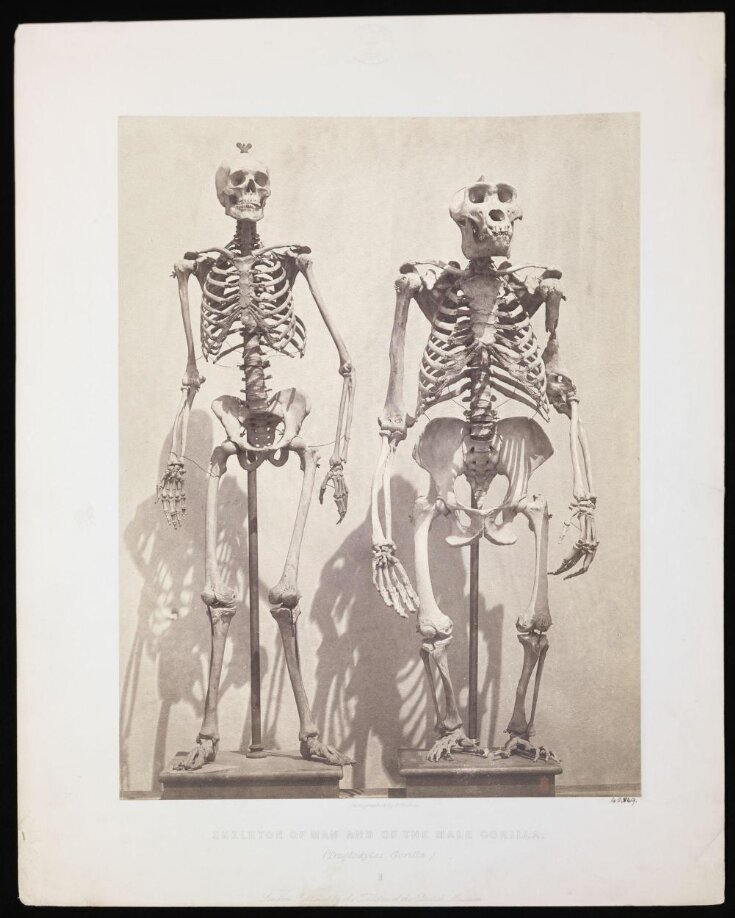This image is a rectangular, matted, black-and-white vintage photograph framed in a creamy background with a black border. The aged photograph, with sepia tones, features two skeletons meticulously displayed in what appears to be a museum setting. 

On the left stands a tall, upright human skeleton, its arms resting straight down its sides. It is supported by a metal rod attached to a stand. To the right, a skeleton resembling a prehistoric human or possibly a gorilla is exhibited. This skeleton has distinctive features: a larger head, wider cheekbones, a broader pelvis, longer arms, and shorter, more bowed legs. It too is supported by a similar metal rod and stand. 

The shadows of both skeletons cast onto the wall behind them, creating a stark contrast that highlights their structures. At the bottom of the photograph, there is some faded writing, barely legible, with the recognizable words "skeleton" and "gorilla" amongst the text. The photograph, though aged and faded, vividly showcases the anatomical differences between the two skeletons.